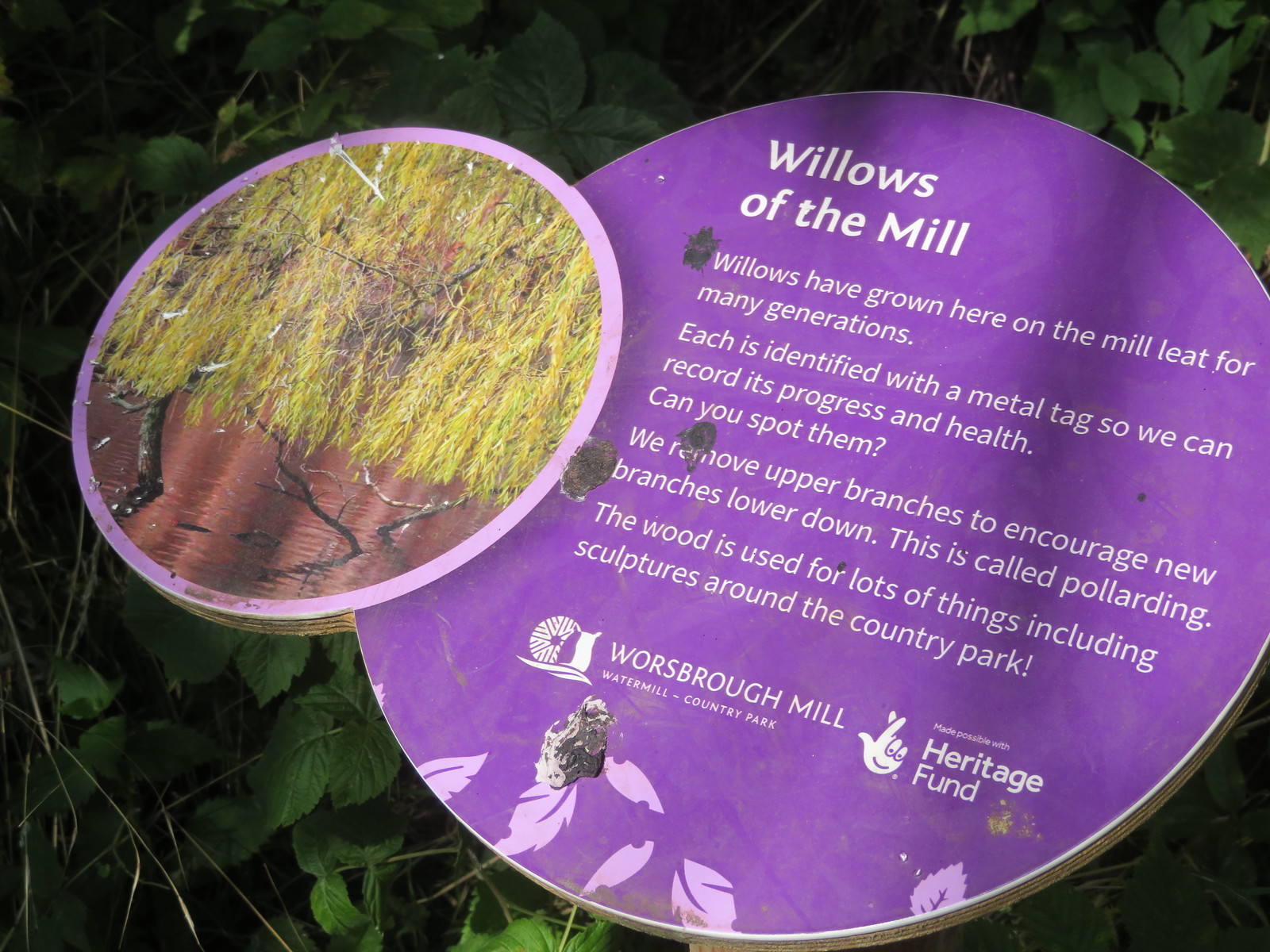The photograph captures an informational placard against a backdrop of dense, shadowy green vegetation. The placard comprises two interconnected circles, with the left circle slightly smaller and bordered in light purple, showcasing an image of a willow tree, which resembles yellow hanging hair. The right circle features a dark purple background adorned with light-colored leaves at its base and white text detailing "Willows of the Mill." The text explains: "Willows have grown here on the mill leet for many generations. Each is identified with a metal tag to record its progress and health. Can you spot them? We remove the upper branches to encourage new branches lower down. This is called pollarding. The wood is used for numerous purposes, including sculptures around the country park. Woodsboro Mill, Watermill, Country Park, made possible with the Heritage Fund."